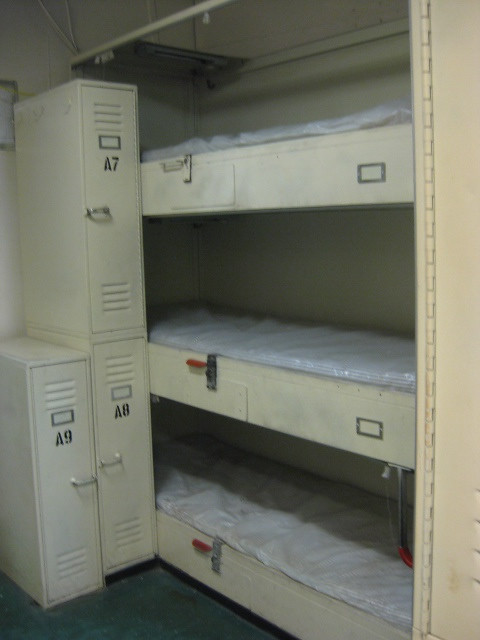This image depicts a cramped and eerie room, likely within a military or naval vessel, or possibly a prison, captured with an older phone. Dominating the scene are three stark, off-white, triple-stacked bunk beds fitted closely against the wall, each with a white plastic-wrapped mattress. These bunk beds, featuring small metal nameplates for identification, offer just enough space to roll over, reinforcing the confined nature of the quarters. The base of the bottom bunk sits directly on the floor, with wooden frames supporting each tier. 

To the left of the bunk beds are three vertically arranged lockers, also in the same off-white color but made of metal. They are labeled with the numbers A9, A8, and A7—A7 being at the top, A8 directly below it, and A9 positioned to the left. The overall atmosphere is accentuated by the dull color palette and the minimalistic, utilitarian design, with a hint of dark green or grey carpet peeking through at the bottom right of the image. The starkness and lack of comfort underscore the functionality of the space, designed for efficiency rather than relaxation.